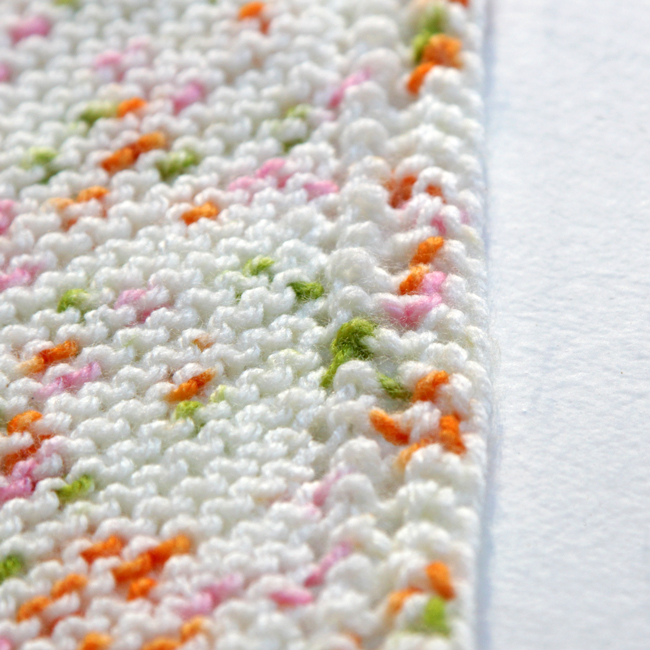This detailed close-up image features a finely knitted or crocheted fabric, likely a blanket or scarf, showcasing a predominant white or creamy-white color. Interwoven throughout the material are vibrant stitches of carrot orange, seaweed green, and a pale pink speckled with darker spots. The fibers display a slight sheen and are meticulously crafted into diagonal rows, suggesting a pattern, although the close-up nature of the photo limits the full design's visibility. The edge of the blanket is visible, bordered neatly, and the entire piece is set against a smooth, white backdrop, possibly another fabric. The blend of colors against the creamy base makes for a striking and potentially very aesthetically pleasing fabric.